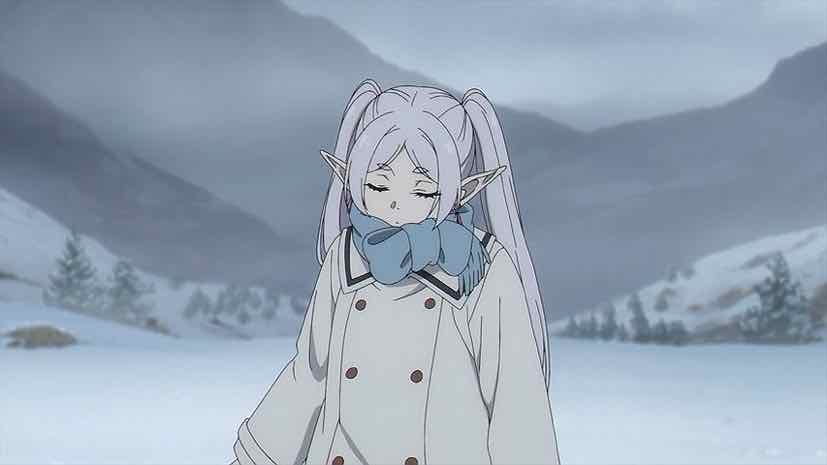This is a detailed description of an anime-style image featuring a female character. The image depicts a winter scene with snow on the ground and dark gray mountainous terrain in the background. The character is centrally positioned, standing outdoors, and dressed in a light gray, tan coat with six buttons visible and a blue scarf adorning her neck. She has long, light gray or purple hair, which drapes over her face and down her back, and her eyes are closed. Notably, she has very long ears. The serene background includes not only mountains but also some green trees interspersed throughout the snowy landscape. The overall color palette consists of muted tones, complementing the wintry theme of the scene.